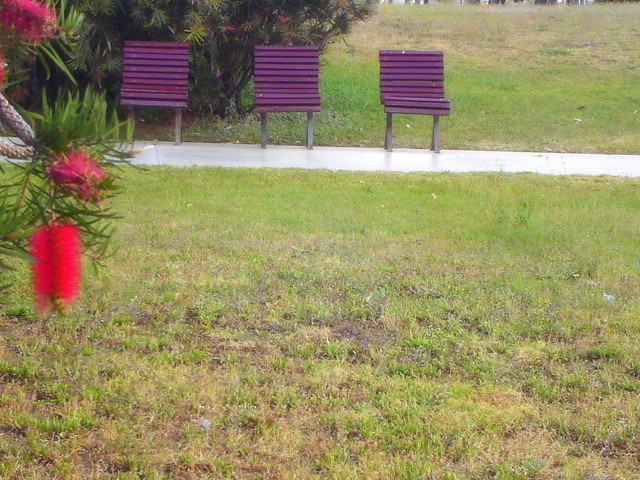This photograph captures a serene park-like setting, characterized by a grassy area that occupies the foreground and bottom two-thirds of the image. The grass appears patchy, interspersed with light green and yellowish-brown strands, and various brown spots of exposed soil, suggesting a transitional season like early spring or possibly after a rain. Dividing the grassy expanse about one-quarter from the top is a smooth, white sidewalk or concrete path, slightly overexposed, which makes its exact texture hard to discern. 

Three evenly spaced, purple one-person chairs with horizontal slats and gray legs sit on this white surface, each separated by about three feet. The legs of these chairs form an upside-down "V" shape, adding a modern flair to the scene. To the left of the sidewalk and chairs, just within the frame, a bush bearing red, cylindrical, bottle brush-like blossoms with spiky leaves protrudes, accompanying a similarly described, partially visible bush on the left edge of the photo. Behind the leftmost and center chairs, an evergreen shrub with red blossoms adds a vibrant backdrop.

The overall atmosphere suggests a tranquil, possibly post-rain setting, with the damp pathway enhancing the fresh, spring-like feel.